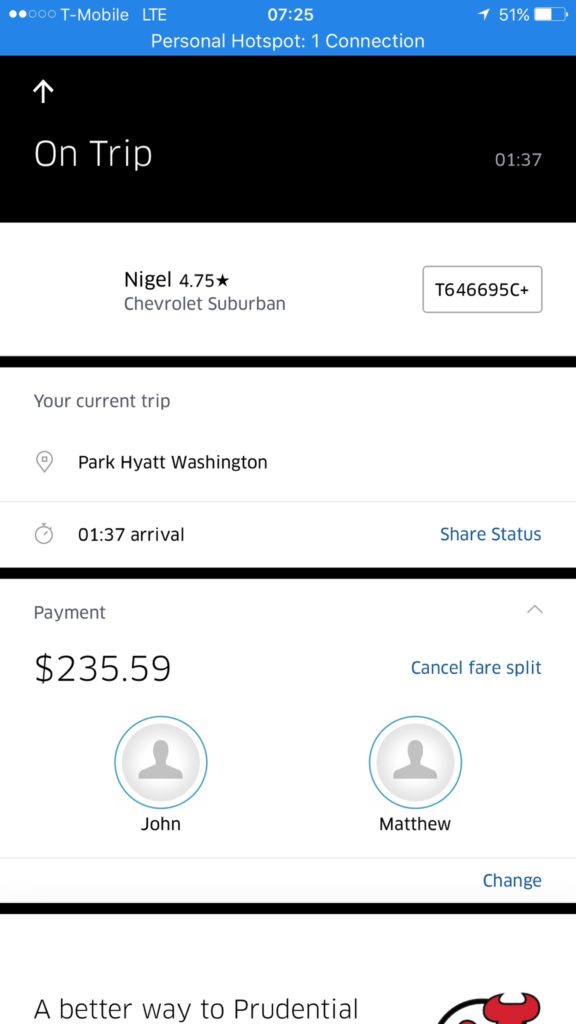In this screenshot, the top portion features a blue banner with white text, displaying "T-Mobile LTE" and the time "7:25" in the center. The battery indicator, showing 51%, is located in the upper right corner. Directly below this banner, there is another blue section centrally stating "Personal Hotspot, One Connection."

Below this, the central portion shows a black box with white text reading "On Trip" on the left and "137" on the right side, set against a white background. Beneath this, the text "NIGEL 4.75" appears, indicating a star rating, followed by "Chevrolet Suburban." Inside a box to the right, it reads "T646695C+."

There is a black horizontal line below this information, followed by a section labeled "Your Current Trip." This part details the destination "Park Hyatt, Washington," with an arrival time of "137." A link for "Share Status," written in blue text, is positioned to the right. 

Further down, another black horizontal line separates the sections. The following part lists "Payment, $235.59." Below this, there are circles representing two people, "John" on the left and "Matthew" on the right.